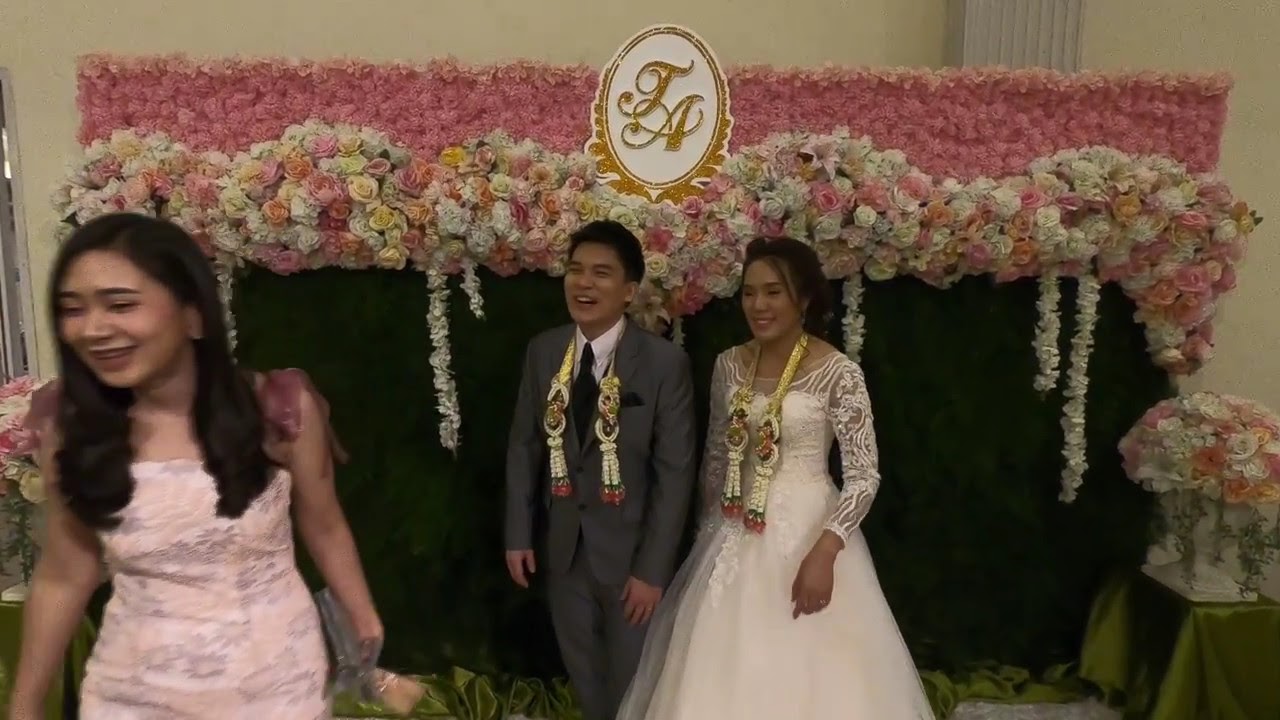In this image, we witness an intimate wedding ceremony set inside a softly lit room with light yellow walls. At the center, an Asian couple stands beaming. The groom, positioned on the left, has dark hair and is dressed in a full gray suit paired with a white shirt and a black tie. Draped around his neck is a celebratory shawl made of gold, white, and pink beads. To his right, the bride, also with dark hair, radiates elegance in a white wedding dress and wears a matching decorative necklace adorned with figures. Surrounding them is an elaborate floral arrangement featuring pink and white flowers with green leaves. Above them, an oval crest with gold-trimmed edges bears the initials "T&A" in gold. To the left of the couple, another woman stands smiling, dressed in a strapless, light pink floral-patterned gown. She too appears to share the same Asian heritage as the couple. Additionally, to the right of the bride, there is a small table covered with a green cloth and topped with a bouquet of flowers, mirroring the floral theme of the room.